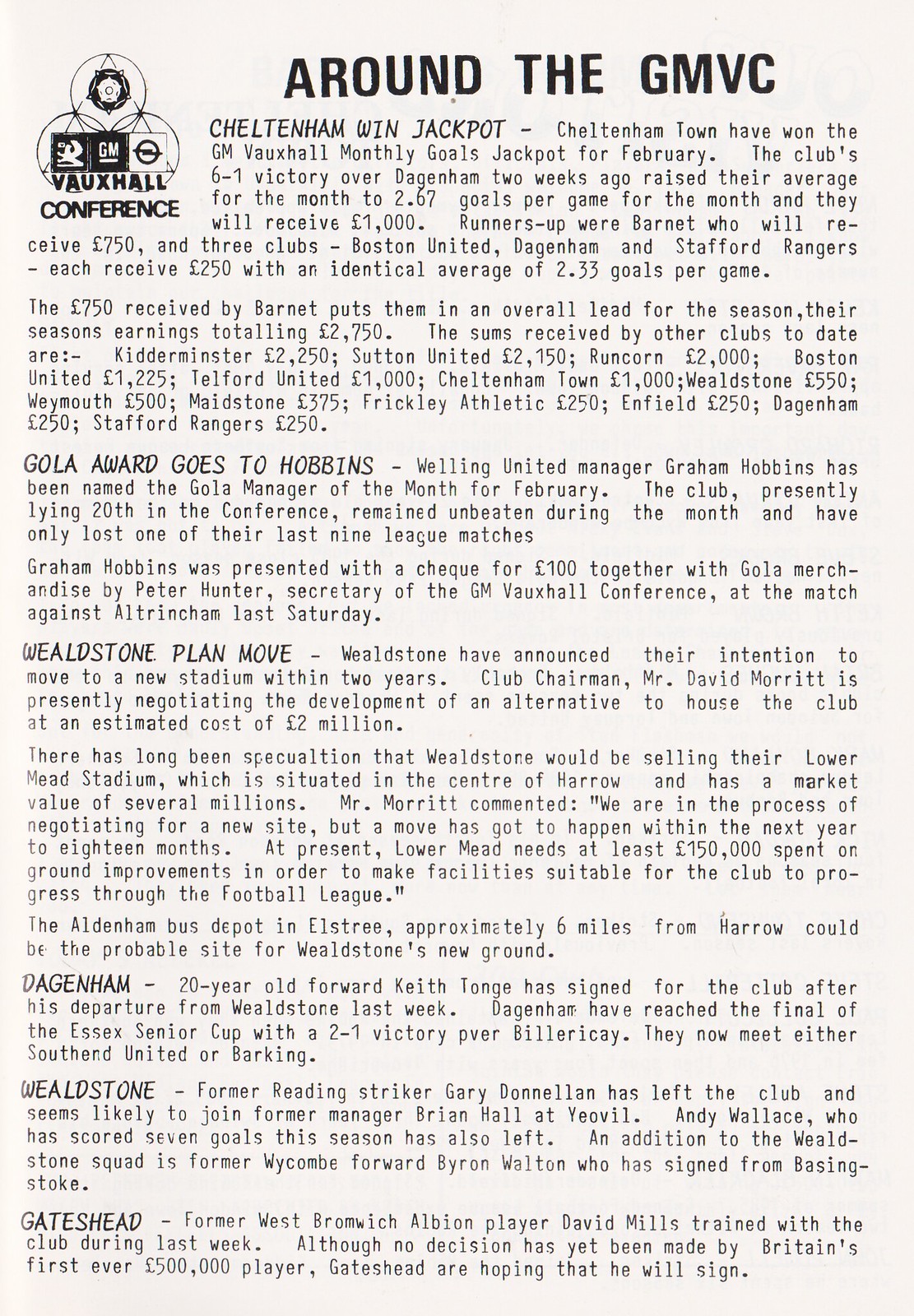The image is a black-and-white vertical photograph displaying a printed piece of paper filled with several paragraphs of text. The title, prominently positioned at the top, reads "Around the GMBC," detailing various clubs winning the monthly goals jackpot. Featured prominently in the text is the success of Cheltenham Town, which won the GMVolhau monthly goals jackpot for February, thanks to a 6-1 victory over Dagenham that pushed their average to 2.67 goals per game. This achievement netted them a prize of £1,000. 

Barnet secured the runner-up position, earning £750, which also propelled them into the overall seasonal lead with total earnings of £2,750. Further down, the text lists that three clubs – Boston United, Dagenham, and Stafford Rangers – earned £250 each, all having an identical average of 2.33 goals per game. An extensive summary of season earnings for various clubs is also provided: Kitterminster with £2,250, Sutton United with £2,150, Runcorn with £2,000, among others. The photograph captures this detailed account set on a standard piece of white paper with black text, typified by its straightforward layout and numerous annotated paragraphs.